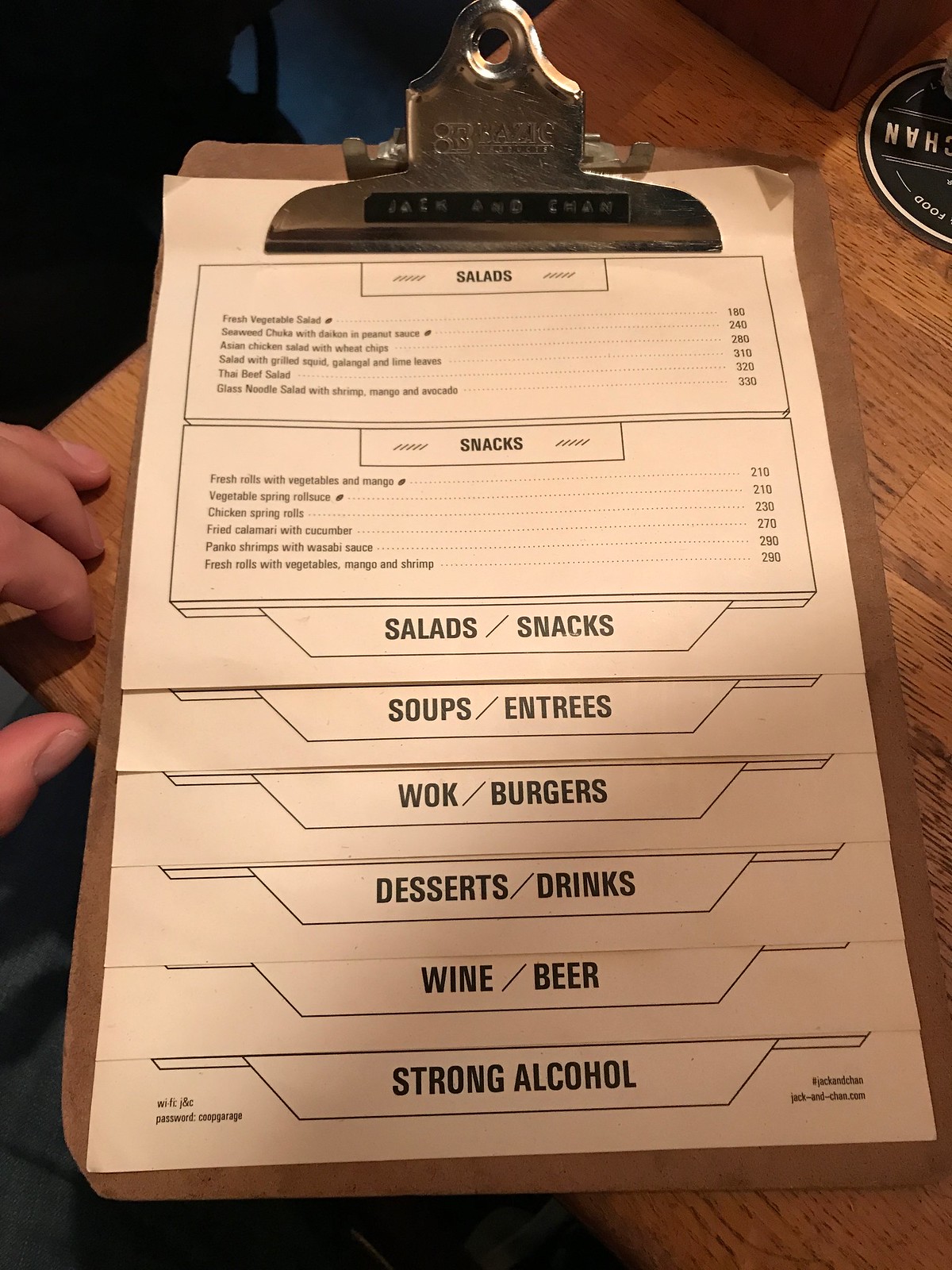This vibrant photograph captures a close-up scene featuring a portion of a left human hand and a clipboard resting on the corner of a desk. The clipboard, adorned with a silver clip, displays a small, plastic, self-printed label, though the text on the label is unreadable. Clipped to the board, a stack of papers, seemingly menus, cascades down its surface. The foremost menu lists items and prices under the headings "Salads" and "Snacks." At the bottom of this menu, a parallelogram contains the text "Salads/Snacks." This pattern continues with subsequent menus peeking underneath, each naming different food and drink categories such as "Soups," "Entrees," "Wok," "Burgers," "Desserts," "Drinks," "Wine," "Beer," and "Strong Alcohol," all aligned in a neat, overlapping row.